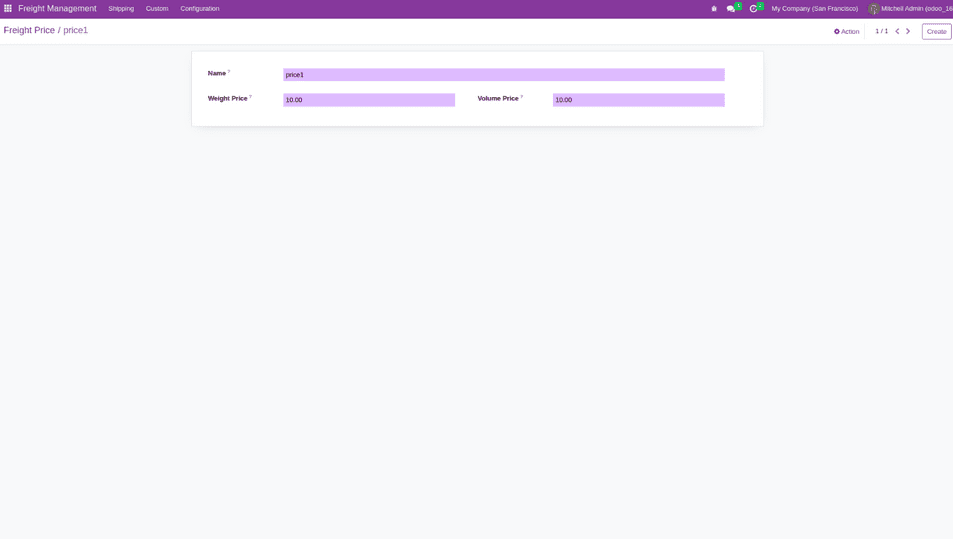The image depicts a website interface with a structured layout. At the top of the page, there is a medium purple to magenta banner that provides a visually appealing header. Within this banner, there is a square divided into three sections, marked by lines on each side. The text inside this square reads "Freight Management" and "Shipping Custom Configuration".

To the right of this square, there are small text bubbles accompanied by a green sign, along with a white circle bearing a green sign at the top. The header area also includes the text "My Company" followed by "San Francisco" in parentheses and "Michael Admin", though part of this is cut off. 

Below the header, there is a white banner featuring the text "Freight Price/Price1" (with "1" being a numeral and the entire phrase written as one word). To the right, the banner includes the label "Action" and an indicator showing "1 of 1" or "1/1," with left and right arrows for navigation. Adjacent to these indicators is a small rectangle outlined in purple, containing the text "Create" written in purple.

Further down, the page displays a long white rectangle. The first section within this rectangle is labeled "Name," featuring a lighter purple rectangle inside, which contains the text "Price 1". Beneath this section, there are additional labels: "Weight Price" with a value of "10.00" and "Volume Price" also with a value of "10.00". The detailed layout and various sections provide a comprehensive overview of the website’s interface and options for freight management.